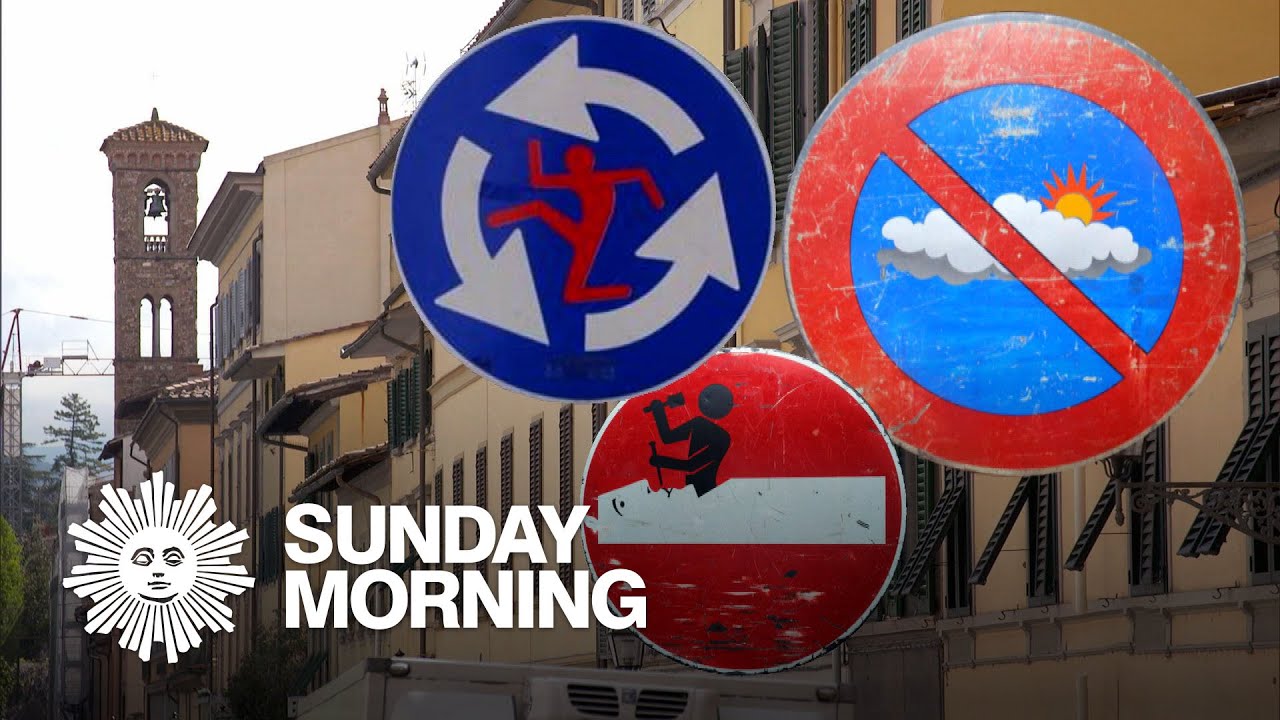This is a color photo advertisement for the CBS television program "Sunday Morning." In the lower left corner, the CBS Sunday Morning logo is prominently displayed, featuring a white illustration of a sun with two eyes, a nose, and a mouth. To the right of the sun, bold white letters spell out "Sunday Morning." 

The background of the advertisement depicts a quaint village or town street, characterized by stone and brick buildings with black shutters. Prominently visible is a church cathedral tower with a bell, various store fronts, and other tan-colored, two to three-story-high structures with brown lines. The sky above is white with clouds.

In front of the storefronts, three distinct circular road signs are visible. The first sign, a blue circle with white arrows, encloses a red figure with arms and legs spread out. Below it, a red circle features a white square and a black silhouetted figure that appears to be holding a microphone or a tool. The last sign, a red circle with a diagonal red line, contains blue clouds and a yellow sunburst, possibly indicating a prohibition of clouds. Additionally, a crane and a partially visible box truck are in the distant background, contributing to the town's active ambiance. This detailed image serves as the setting for highlighting the Sunday Morning program.